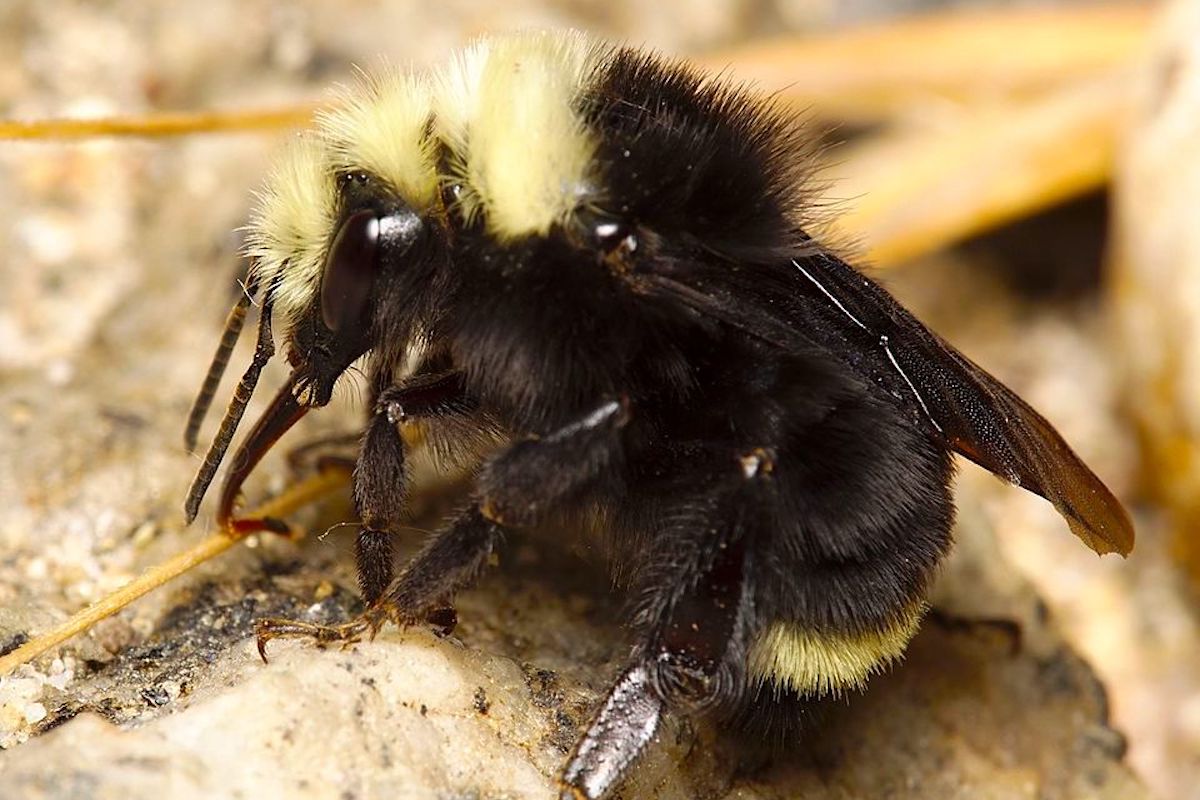The image is a close-up, landscape-oriented color photograph of a bumblebee, showcasing detailed realism. The bee, positioned in profile with its head in the top left and tail towards the bottom right, is captured in exquisite detail. Its thick, fuzzy fur coat, predominantly black with distinct yellow markings, covers its head, shoulders, and part of the abdomen. The yellow fur is particularly noticeable around the top of the back, head, and a band midway down the tail. The bee's black eyes and segmented legs, which appear shiny in the natural sunlight, are also clearly visible. Its antennae hang down, and its wings, showing hints of deep red and white, are folded back over its body. The background is a soft, gold-colored, out-of-focus surface that could be a pale, light brown log, stone, or beach driftwood. The natural light from the right side enhances the intricate details of the bee, creating a striking representation of its texture and color.